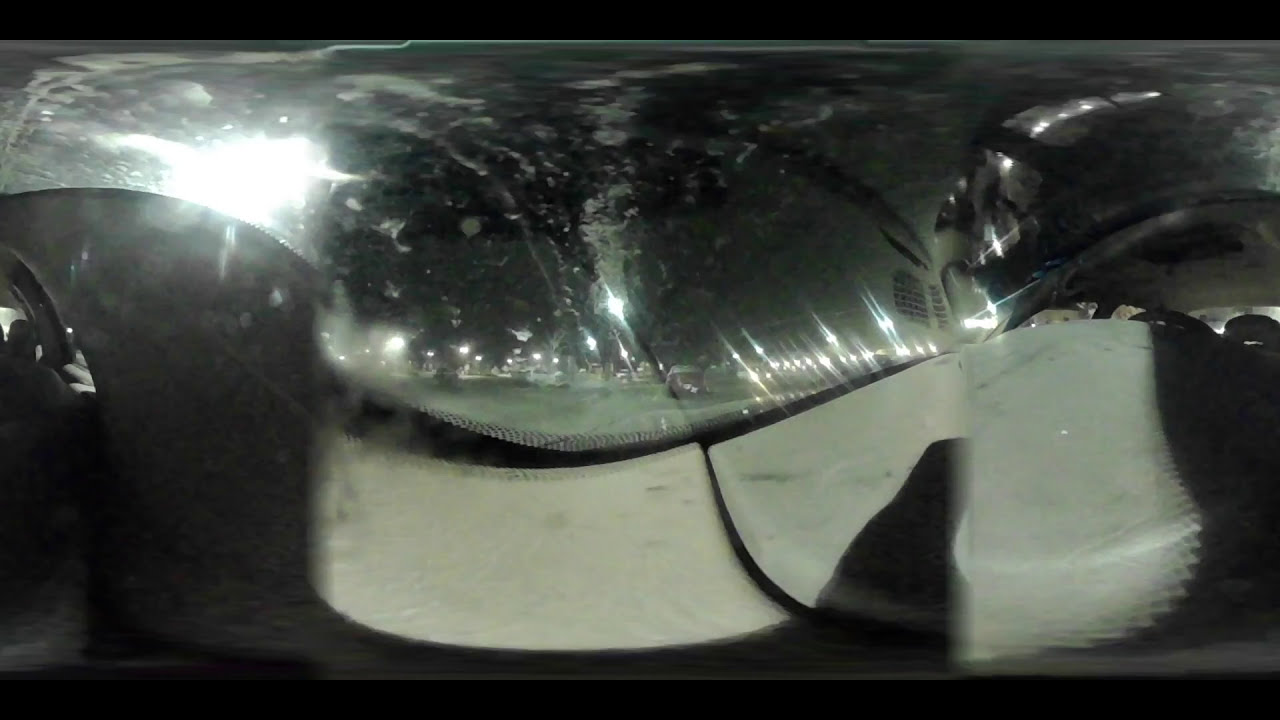In the center of this distorted, wide rectangular image, taken from what appears to be inside a vehicle or through a windshield, lies a peculiar white object resembling a shoe with a long heel, leaning down to the left and split in half near the base. The overall texture and form of this central object evoke the appearance of a piece of clay. The high curvature of the angles in the image suggests a panoramic or lens-distorted photograph. The surface above the object resembles a dirty windshield marked by numerous water streaks, with light scattering from the upper left to the bottom right. In the top left corner, a bright white light pierces through the glass, dramatically illuminating the scene. Black strips frame the top and bottom of the image, giving it a cropped, cinematic feel. The background reveals an expanse of gray concrete with several distant white lights, hinting at an outdoor setting, possibly a road with cars. The entire scene is viewed through a grimy window that distorts colors into shades of black, white, gray, yellow, and hints of light green, contributing to the low quality and blurry appearance of the photograph.